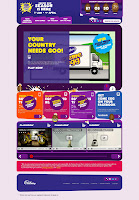This image is a blurry screenshot of a vibrant website or app interface. At the top, an eye-catching fuchsia background frames a dark blue header with rounded corners. Within this header, white text is positioned at the top left, accompanied by a yellow figure. Below this section, four purple tabs display white text.

To the right of the header, a prominent purple rectangle contains four brown characters. The first three characters have distinct white eyes, while the fourth character does not.

Moving down the page, a large section features a cartoon image of a white box truck driving along a gray road with a green hill in the background. This image is accented by a blue badge in the top right corner. Overlapping this picture on the left half is a purple translucent overlay with yellow text that reads, "Your country needs goo." A mint green mat with a black interior border also frames the truck image.

Below this, four sections of colored, offset rectangles with rounded corners appear, arranged horizontally from left to right. The rectangles are orange with white text, red with white text, purple with white text, and blue with white text. The first three of these sections feature additional purple badges with intricate yellow and white designs.

At the very bottom, the screenshot shows another section characterized by a purple background. This area contains three videos, each marked with a silver play button in the center, ready for interaction.